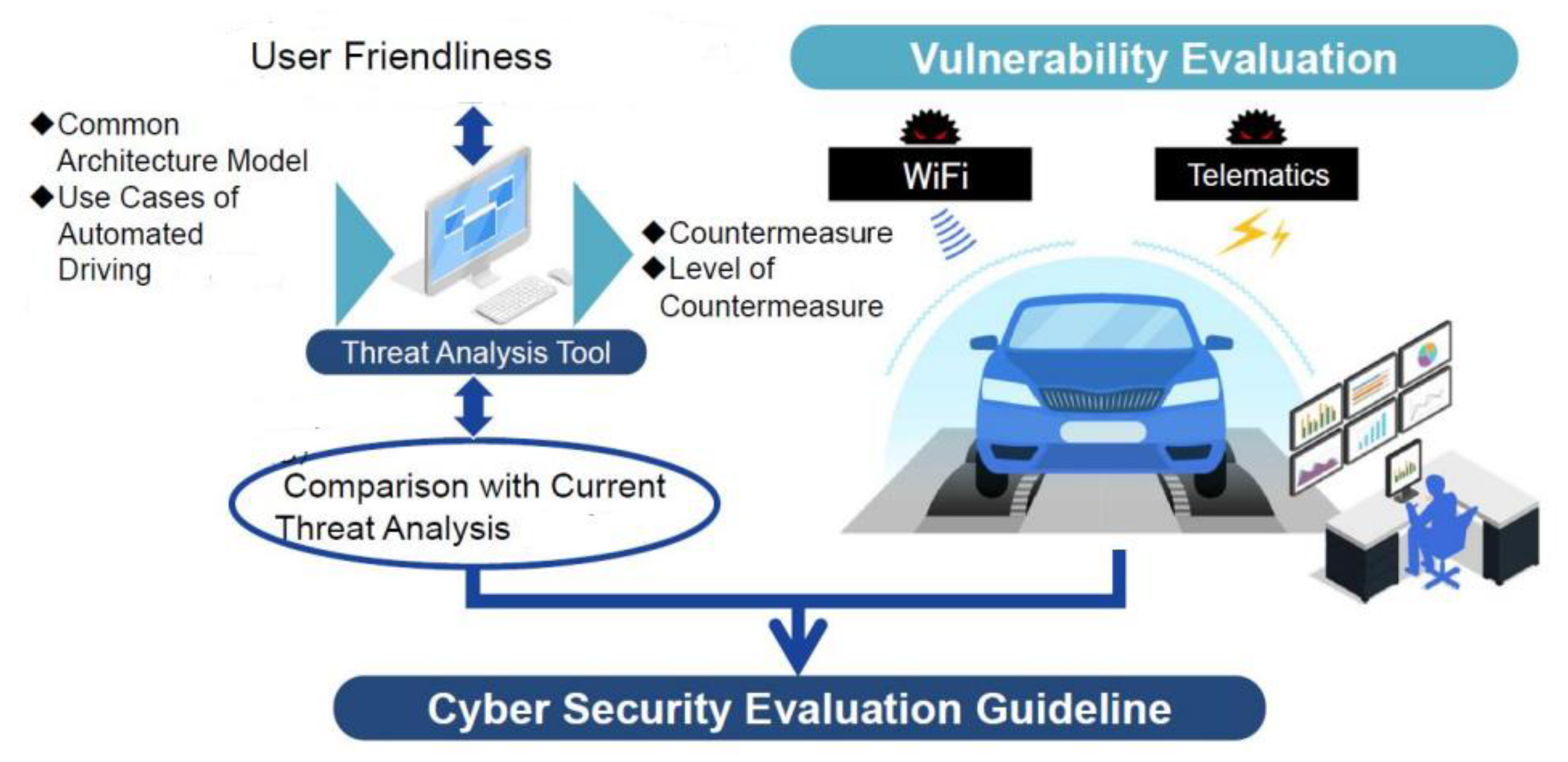The image is a detailed infographic titled "Cybersecurity Evaluation Guide" positioned at the bottom, structured as a comprehensive flowchart for assessing self-driving car security. At the top, the title "Vulnerability Evaluation" is prominently displayed. On the top-left corner, there is a section labeled "User Friendliness," pointing to a computer monitor and keyboard. To the left of this monitor, there are bullet points listing "Common Architectural Model" and "Use Case of Automated Driving." On the right side of the monitor, additional bullet points read "Countermeasure" and "Level of Countermeasure," with the monitor labeled "Threat Analysis Tool." An arrow from this tool points to a blue oval labeled “Comparison with Current Threat Analysis.”

An arrow descends from the oval to a sign on the right that reads "Cybersecurity Evaluation Guide," which is next to an illustration of a blue car on a gray street. Above the car, two rectangles display "Wi-Fi" and "Telematics." Additionally, there's a label above these rectangles stating "Vulnerability Evaluation."

At the bottom-right of the image, near the car, there is a depiction of a person sitting at a desk working on a computer with a chart displayed on the screen. Surrounding the person are six frames on the wall, each containing various charts—bar charts, pie charts, and line charts in different colors.

The image consistently uses a color scheme of blue, black, and white for text bubbles and various graphical elements, providing a cohesive and visually organized illustration of cybersecurity measures for autonomous vehicles.